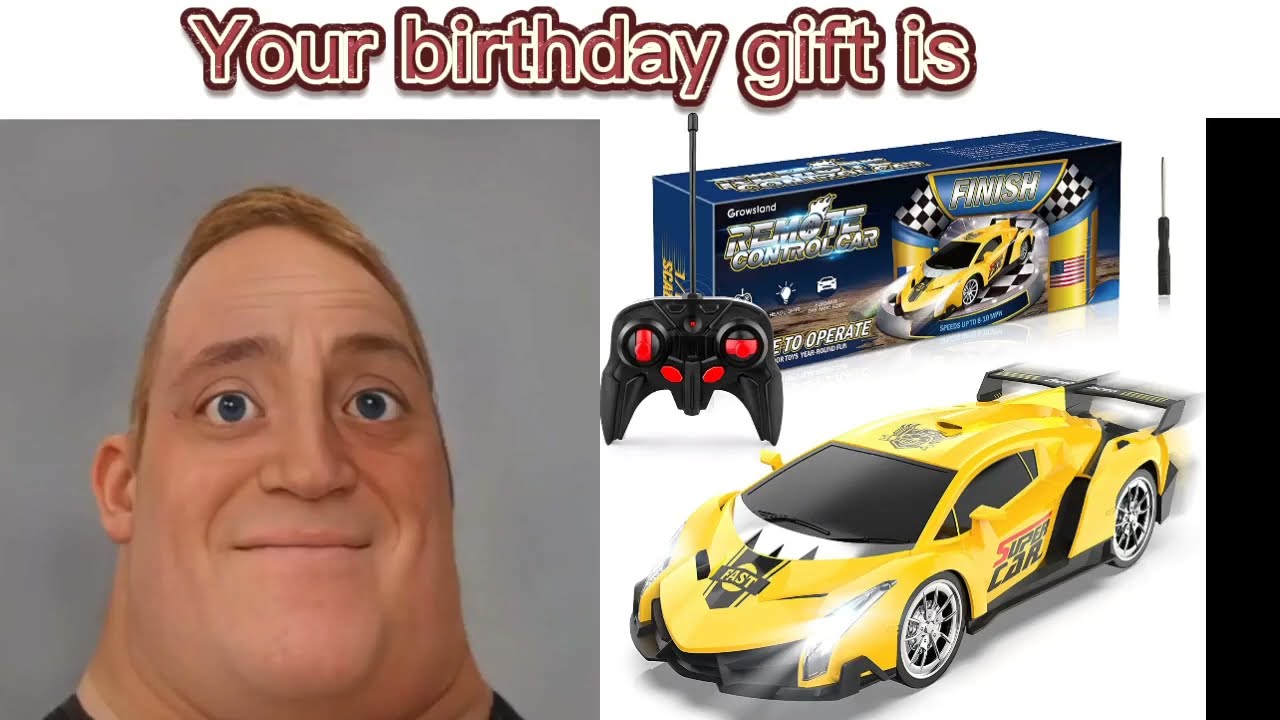The image consists of two separate pictures stacked side by side with the text "Your Birthday Gift Is" displayed above them. The text is brown, bordered first by white and then by black, all set against a white background. The picture on the left features a three-dimensional cartoon-style man with a distinctively exaggerated head and face. The character, reminiscent of a modified Mr. Incredible from Pixar's "The Incredibles," has short blonde hair, large blue eyes, and a conspicuously wide neck and cheeks, giving his face a stretched and goofy appearance. His mouth, marked by pink lips, is a straight line, adding a subtle smile due to his accentuated cheeks. The image on the right showcases a yellow remote-controlled race car with the word "Fast" written on its hood and "Supercar" on its side. The car features a spoiler and is presented alongside its packaging, which includes a black remote control with red buttons and a small screwdriver.